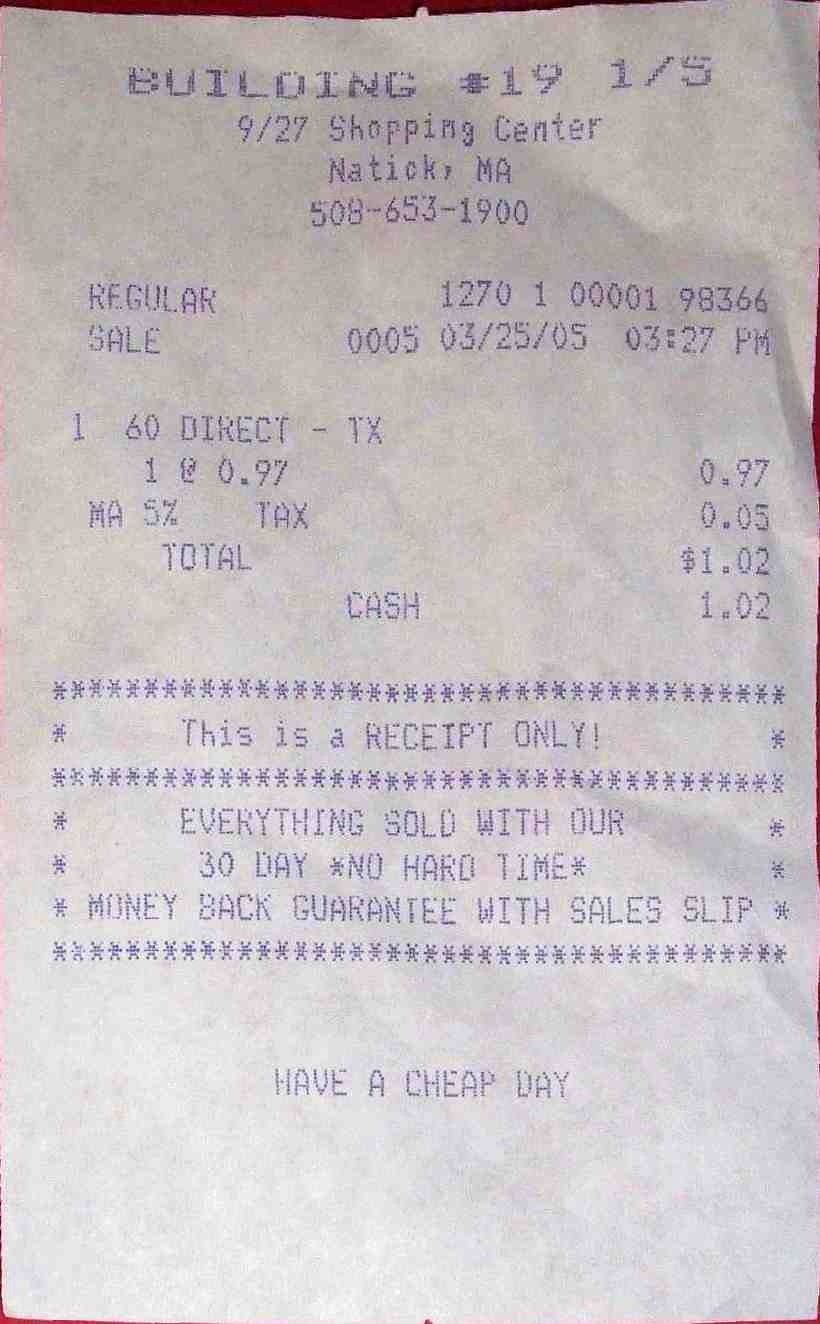The image shows a vertically taken photo of a white paper receipt with dark blue faded text. At the top center of the receipt, it reads "Building 19, 1-5, 9-27 Shopping Center, Nattick, Massachusetts." Below this, it provides a phone number: "508-653-1900." The receipt also shows several identifier numbers and timestamps, with one column on the left and corresponding details on the right. It reads "Regular Sale" followed by a string of numbers, "127010000198366," and the date and time "05/03/25, 03:27pm." The receipt is for "1, 60 Direct, Texas" priced at $0.97, with Massachusetts state tax of 5 cents, bringing the total to $1.02, paid in cash. Towards the bottom, the receipt emphasizes that it is "a receipt only" and mentions that "everything sold comes with a 30-day no-hard-time money-back guarantee with sales slip." Framing these details are rectangles drawn with star symbols. The receipt concludes with "Have a cheap day" in the bottom middle.